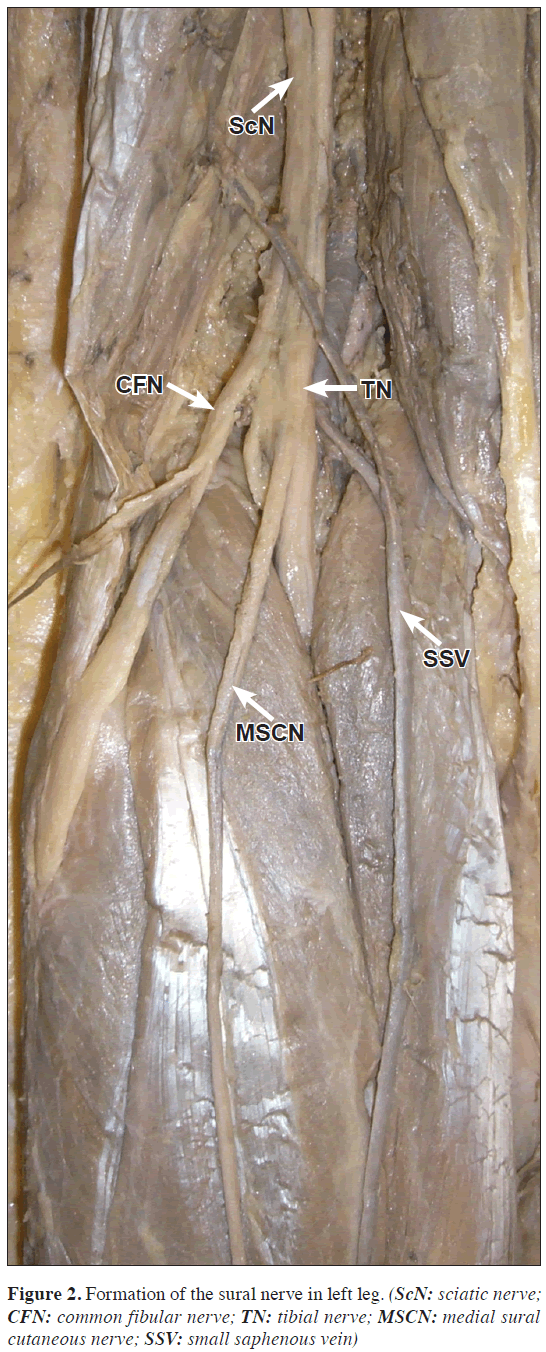The image depicts a detailed view of the interior of a human leg, focusing on the various nerves and veins. The primary colors range from light brown to dark brown, with the tissue appearing gray and beige. Protruding from the muscular structure are several nerves, each annotated with arrows and labeled with abbreviations.

At the top of the image, a white arrow points to the "SCN" (Sciatic Nerve), while another arrow points to "CFN" (Common Fibular Nerve). "TN" (Tibial Nerve) is indicated by an arrow pointing to the left, and "MSCN" (Medial Sural Cutaneous Nerve) sits in the middle with an arrow pointing up and to the left. "SSB" (Small Saphenous Vein) is labeled on the right with an arrow also pointing up and to the left. 

The bottom of the vertical rectangular image features a white horizontal section with small black text that reads: "Figure 2, Formation of Sural Nerve in Left Leg," followed by a bracket listing all the labeled parts and their corresponding full names:
- SCN: Sciatic Nerve
- CFN: Common Fibular Nerve
- TN: Tibial Nerve
- MSCN: Medial Sural Cutaneous Nerve
- SSB: Small Saphenous Vein

This comprehensive annotation aids in identifying and understanding the intricate network of nerves within the leg.